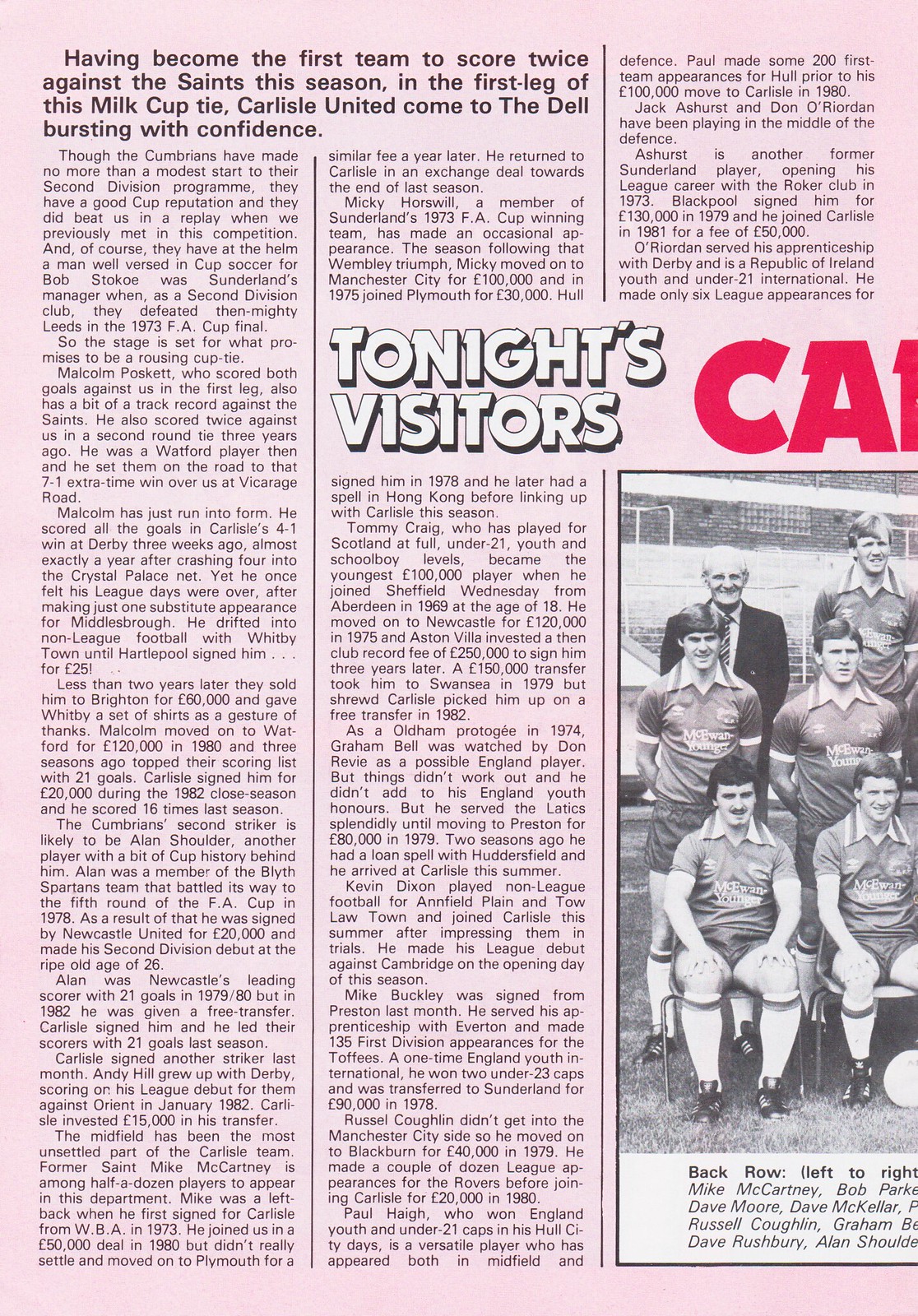This detailed photograph captures a page from a soccer magazine, prominently featuring an article set against a very light pink background. The upper left-hand corner of the page displays the title of the article in bold black text, which reads, "Having become the first team to score twice against the Saints this season in the first leg of this Milk Cup tie, Carlisle United come to the Dell bursting with confidence." The text continues into three columns. 

In the middle column, bold white text states, "Tonight's Visitors," while red text next to it begins with the letters "C" and "A," suggesting it's a cut-off part of a team name or title. The article details a rich history involving both teams and specific players, emphasizing Carlisle United's formidable form and notable players such as Malcolm Poskitt and Alan Shoulder, both known for their impressive track records and significant contributions in previous matches and seasons.

At the bottom of the rightmost column, there's a black and white photograph partially visible. This image shows a soccer team posing for a photo; the players in the back are standing while those in the front are seated. An older man in a suit and tie, probably the coach, is also visible. The photo extends beyond the page, indicating it continues onto the next part of the magazine.

Overall, this page blends a historic commentary with visual elements, highlighting key players, team dynamics, and an atmosphere of anticipation for a thrilling cup tie match.